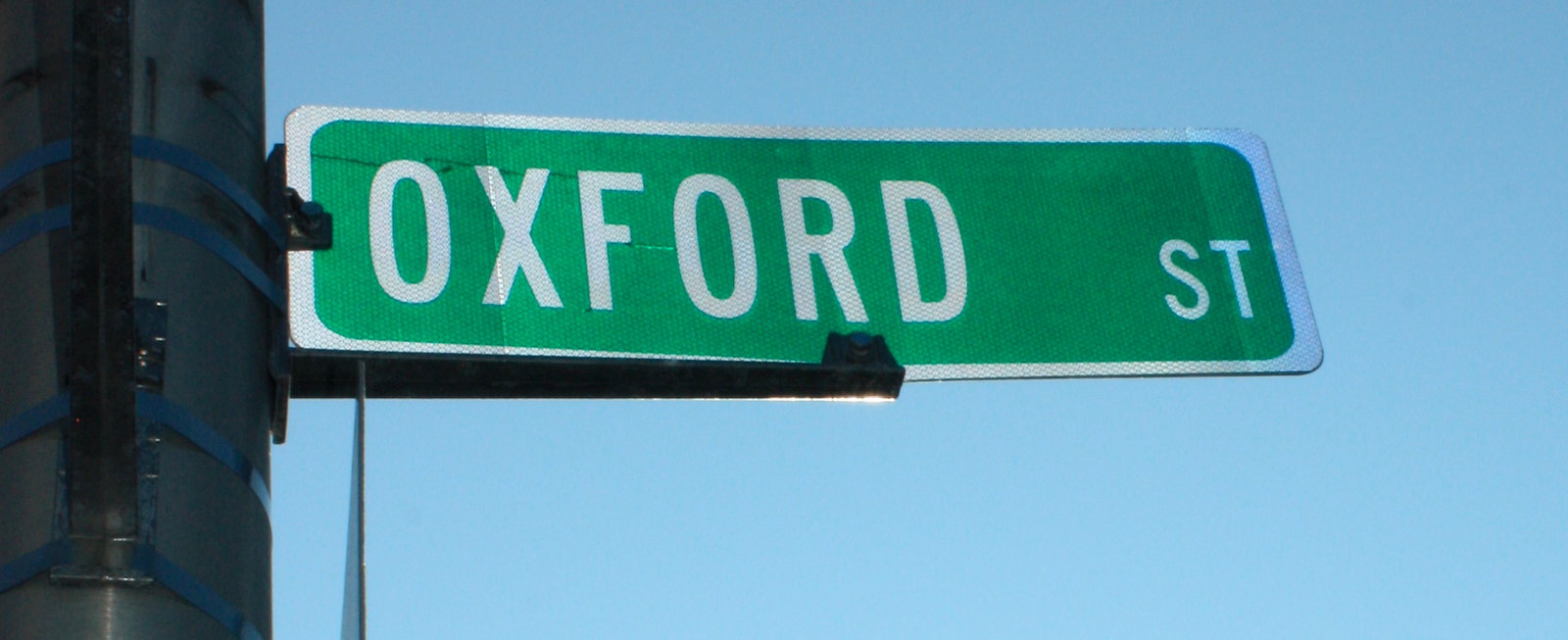This color photograph provides a close-up view of a street sign. The sign is mounted on a grayish pole which features dark blue straps wrapped around it. Extending from the left side of the image, the pole contrasts against a beautiful, cloudless blue sky on the right. The street sign itself is green with bold white letters reading "Oxford ST." The sign is outlined in white, making the text stand out sharply. Just below the sign, a metal arm is visible, securing the sign to the pole. The clear sky and detailed textures of the pole and sign create a striking, vivid scene.